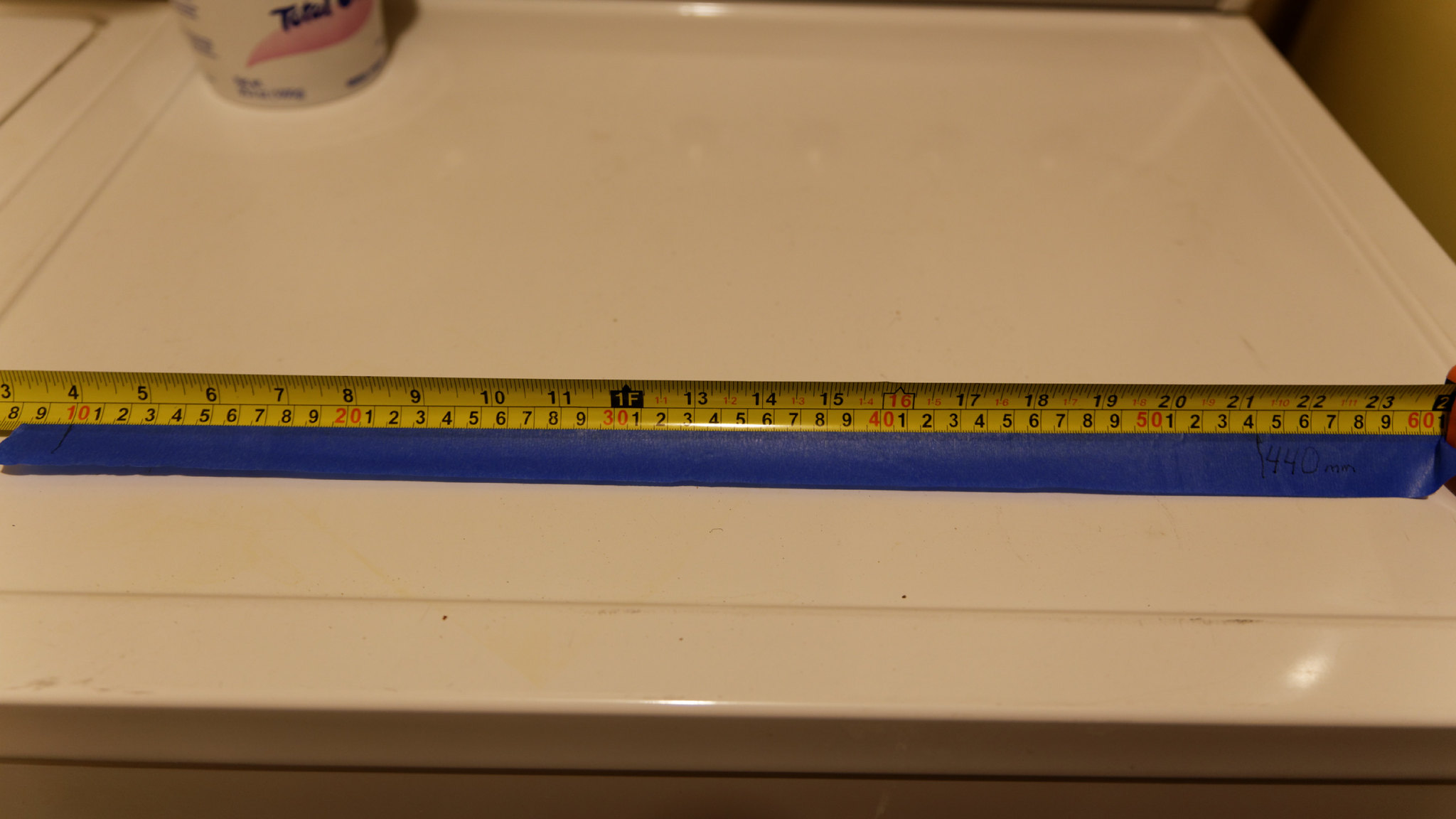The image depicts an indoor scene focused on a white clothes dryer being used as a makeshift work surface. Stretching horizontally across the top of the dryer is a yellow measuring tape, extending from 3 inches to 24 inches. Below the measuring tape lies a strip of blue painter's tape, marked near its end with the measurement "1440 millimeters." Adjacent to the dryer, in the top left corner of the frame, is the lid of a top-loading washing machine. Atop the dryer sits a small white container with a pink swirl and an indistinct label, likely a laundry product such as detergent or bleach. The dryer surface is illuminated by a light source, casting a slight sheen across its top and bottom edges.